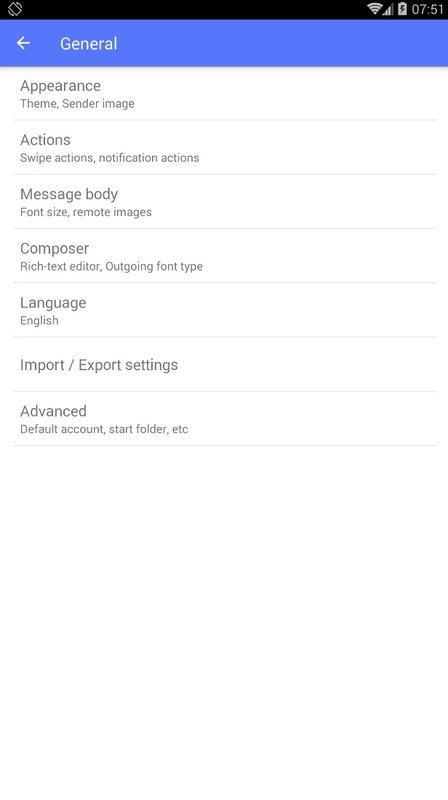The image is a phone screenshot displaying a settings menu. The top right corner shows it is 7:51, with a vertical battery icon next to it, indicating the phone is currently charging through the lightning symbol. To the left of the battery icon, the Wi-Fi signal strength is at three out of four bars, and further left, the phone signal strength shows full bars. On the top left, there's an icon depicting a phone being turned sideways.

Below this status bar, the word 'General' is prominently displayed in white text, accompanied by a leftward arrow icon pointing towards it. Under the 'General' label, several categories are clearly listed on the left side of the screen.

The categories and their respective options are as follows:
1. **Appearance:**
   - Theme
   - Sender Image

2. **Actions:**
   - Swipe Actions
   - Notification Actions

3. **Message Body:**
   - Font Size
   - Remote Messages

4. **Composer:**
   - Rich Text Editor
   - Outgoing Font Type

5. **Language:**
   - English

6. **Import/Export Settings**

7. **Advanced:**
   - Default Account
   - Start Folder